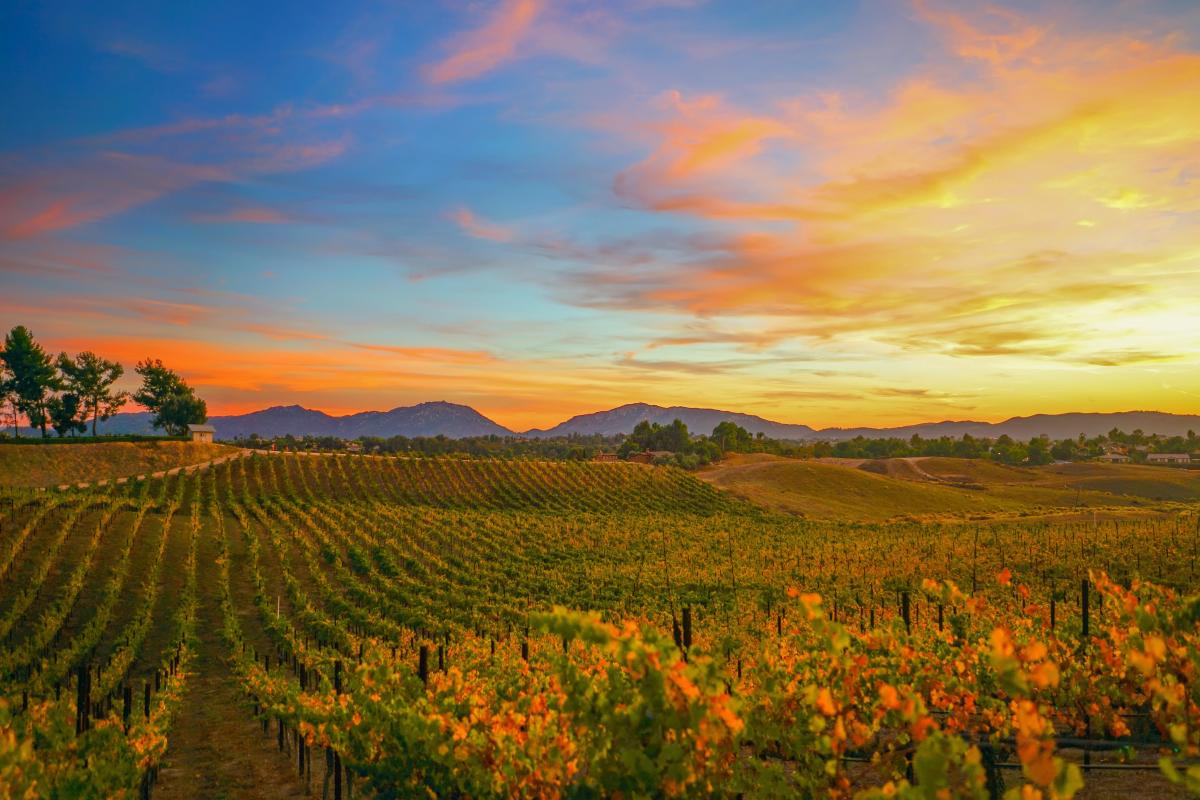This image, a highly realistic painting, captures a breathtaking outdoor sunrise scene. The foreground features meticulously groomed rows of orange five-petaled flowers, which appear to be crops. These vibrant flowers, with their green petals and stems, extend towards the horizon, creating a lush tapestry of color. Each row is carefully delineated, with the crops overlapping over subtle hills. 

In the midground, near the base of tall, rounded mountains, stands a row of green trees providing a natural border between the fields and the distant peaks. The mountains, which have a subtle purple hue, stretch across the horizon. Some small houses are visible on the right-hand side, adding a touch of human presence.

Above the mountains, the sky is a spectacular display of colors. It transitions from bright blue in the upper left corner to a warm yellow as it approaches the horizon, with hints of orange and yellow reflecting the rising sun. Wisps of clouds in the upper right corner catch the golden hues, further enhancing the scene's vividness. This lifelike painting masterfully blends the natural elements, creating an immersive and serene landscape.